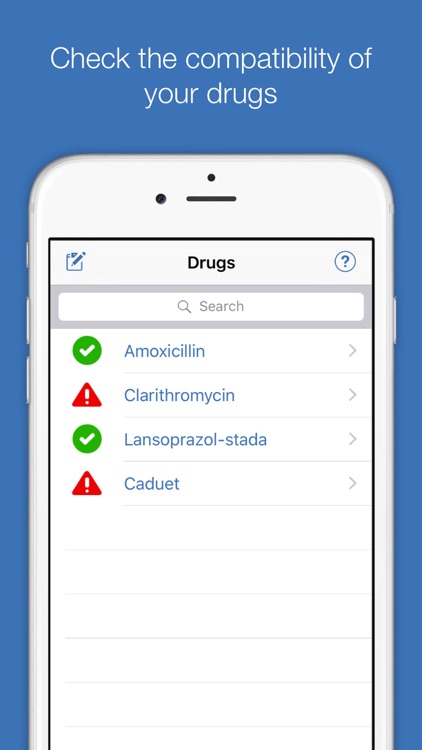A detailed mock-up image of a drug compatibility check application. The top portion of the mock-up features a large blue box with white text that reads, "Check the Compatibility of Your Drugs." The phrase "Check your compatibility of" is on one line, while "your drugs" appears on another. Below the heading, there is an outline of a smartphone on a white background. The phone screen shows some information at the top, with the word "Drugs" centered on the left side. Next to it is a blue icon depicting a pad with a pencil, and on the right side, there is a blue circle with a white question mark inside.

Below this, a long, elongated search box can be seen. The search box has a magnifying glass icon and the word "search" written in light gray text. Further below, the screen displays four rows of information.

1. The first row features a checkbox, a Korean text label, the drug name "Amoxicillin" spelled as "A-K-E-M-O-X-I-C-I-L-L-I-N," and a gray arrow to the right.
2. The second row illustrates a warning triangle with a white exclamation mark inside and the drug name "Clarithromycin" spelled as "C-L-A-R-I-T-H-R-O-M-Y-C-I-N."
3. The third row contains a checkbox with Korean text and the drug name "Lansoprazole" misspelled as "L-A-N-S-O-P-R-A-Z-O-L-D-A-S-T-A-T-A."
4. The fourth row shows another warning triangle with a white exclamation mark and the text "CATUET."

The detailed layout and use of symbols make it easier for users to identify compatibility issues with their medications.